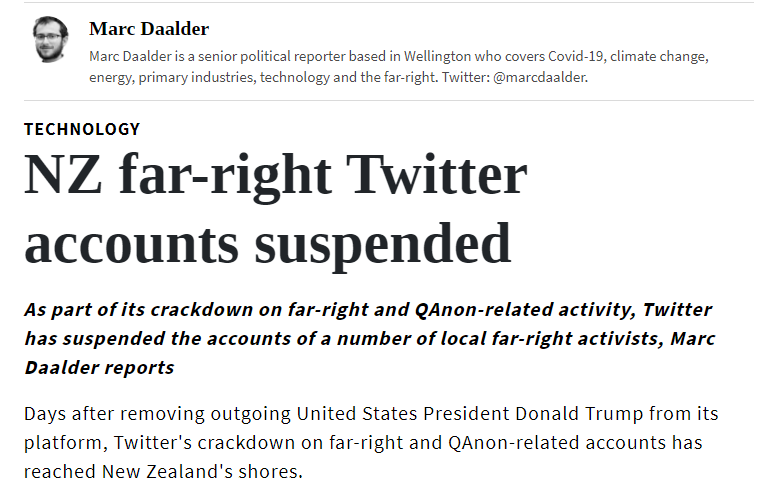The image features an excerpt from a publication by Mark Dalter, a senior political reporter based in Wellington. Dalter specializes in covering various topics including COVID-19, climate change, energy, primary industries, technology, and the far right. His Twitter handle is @MarkDalter. 

The excerpt highlights a significant development in social media regulation: the suspension of New Zealand far-right Twitter accounts. This action is part of Twitter’s broader effort to crack down on far-right and QAnon-related activities. The suspension of these local accounts follows closely on the heels of Twitter’s decision to remove outgoing U.S. President Donald Trump from its platform. 

The headline "NZ far right Twitter accounts suspended" is prominently displayed in bold black text on a white background, emphasizing the gravity of the report. The detailed narrative underscores Twitter's global initiative to regulate and mitigate extremist content.

Overall, the image encapsulates the ongoing efforts to maintain digital safety and standards through the regulation of far-right activities on social media platforms.